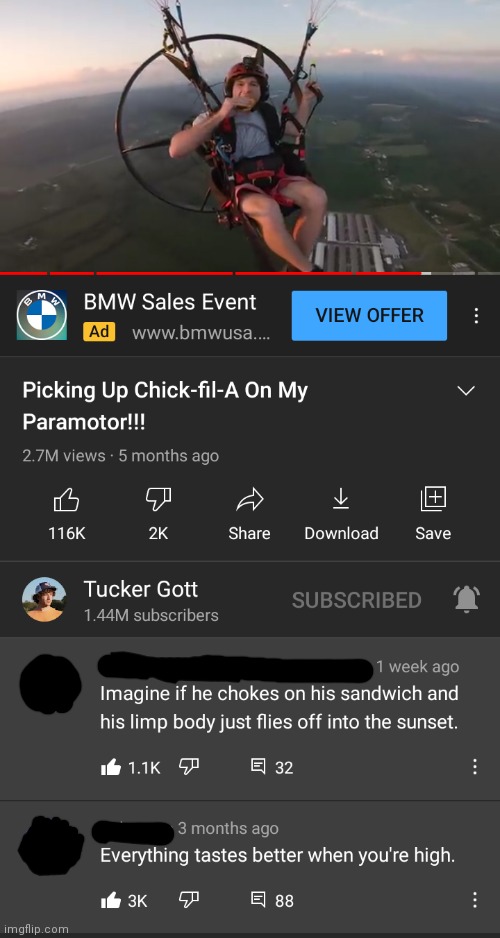Screenshot from a BMW USA sales event promotion. The image features a person named Tucker, who is depicted sitting in an unconventional manner as if floating in the sky, giving the impression of a parachute-like posture. He appears to be part of an imaginative scenario, with a surreal suggestion that his body might separate and fly off into the sunset if choked on a sandwich. The visual is highly engaging, as evidenced by its popularity—garnering 116,000 likes. Tucker's substantial influence is highlighted by his 1.8 million subscribers. The event is underscored by the iconic BMW emblem, reinforcing the brand's presence. The screenshot, with its blend of whimsy and brand elements, captures attention and stirs curiosity.